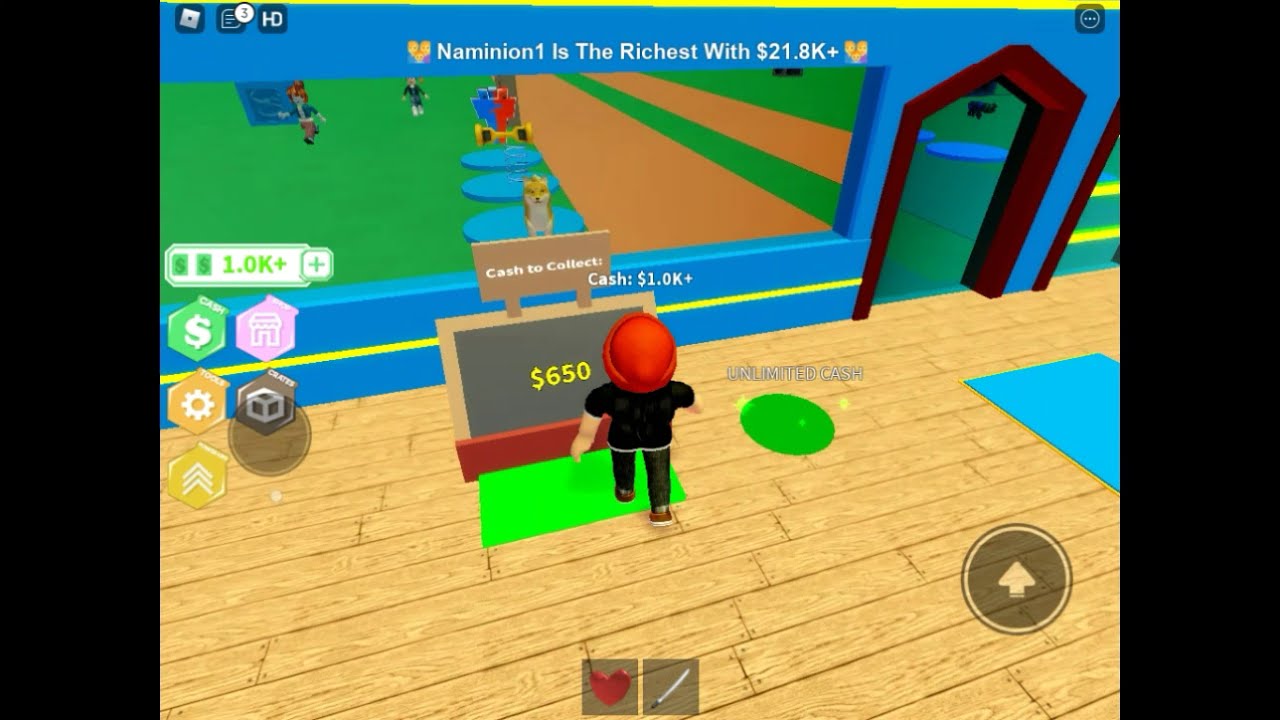This horizontal rectangular image, presumably a screenshot from a computer game, features a digital scene framed by thick black borders on the left and right, making the central colorful part appear almost square. Centrally positioned is the backside of an avatar with brown hair, dressed in a black short-sleeved shirt, black pants, and an orange cap, who is stepping onto a bright green rectangular spot on the wooden floor. The figure stands before a chalkboard-like screen displaying "$650" in yellow, with "Cash to collect" written above in white letters. The backdrop features a blue wall adorned with yellow horizontal stripes and a doorway in the upper right corner leading into another room. To the left of the avatar, a window reveals a grassy area with small blue circular shapes, likely representing people, surrounded by pathways. The upper portion of the scene contains text declaring "Namination 1 is the richest with $21.8K," and beside it are three hexagonal icons. Additionally, the left side displays another set of five hexagonal icons including a dollar sign, amounting to "1.0K+" in green. The bottom right corner includes a circle containing an up arrow.